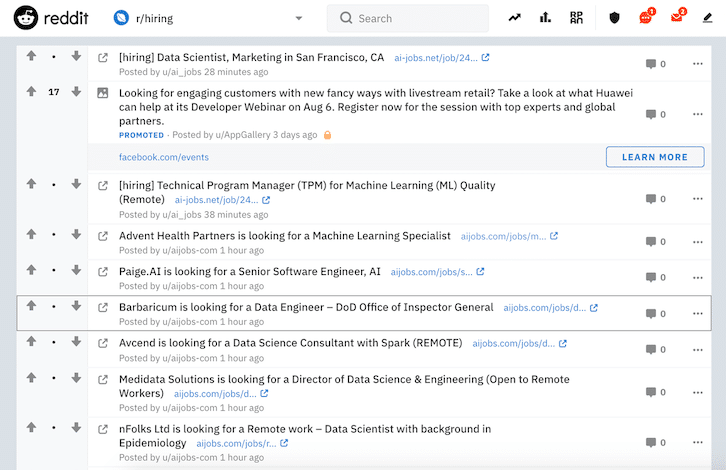This is a detailed screenshot of a Reddit page interface. 

In the upper left-hand corner, there is a black Reddit icon. To the right of the icon, the word "reddit" appears in black lowercase letters. Adjacent to this, there is a white circle with an indistinct white object inside it, followed by the text "r/hiring" in black. Further to the right, there is a black downward-pointing triangle icon. Next to the triangle, there is a gray search bar featuring a magnifying glass icon and the placeholder text "Search." 

Directly below this toolbar, there is a rectangular area outlined with a thick, gray border. On the left side of this rectangle, there is a vertical sequence of upward-pointing arrow icons, extending from top to bottom. Beside the arrows, the number 17 is listed on the second line, while the remaining lines display dots. To the right of these number and dot indicators, there is a column of downward-pointing arrow icons.

To the right part of the main content area, a series of white rectangular boxes are displayed, each containing individual messages. On the right side of each message box, there is a file icon. To the right of the file icon, a zero is displayed, indicating no interactions or counts. Furthermore, at the far right of each message box, there are three horizontal dots arranged to form an ellipsis, suggestive of additional options or settings.